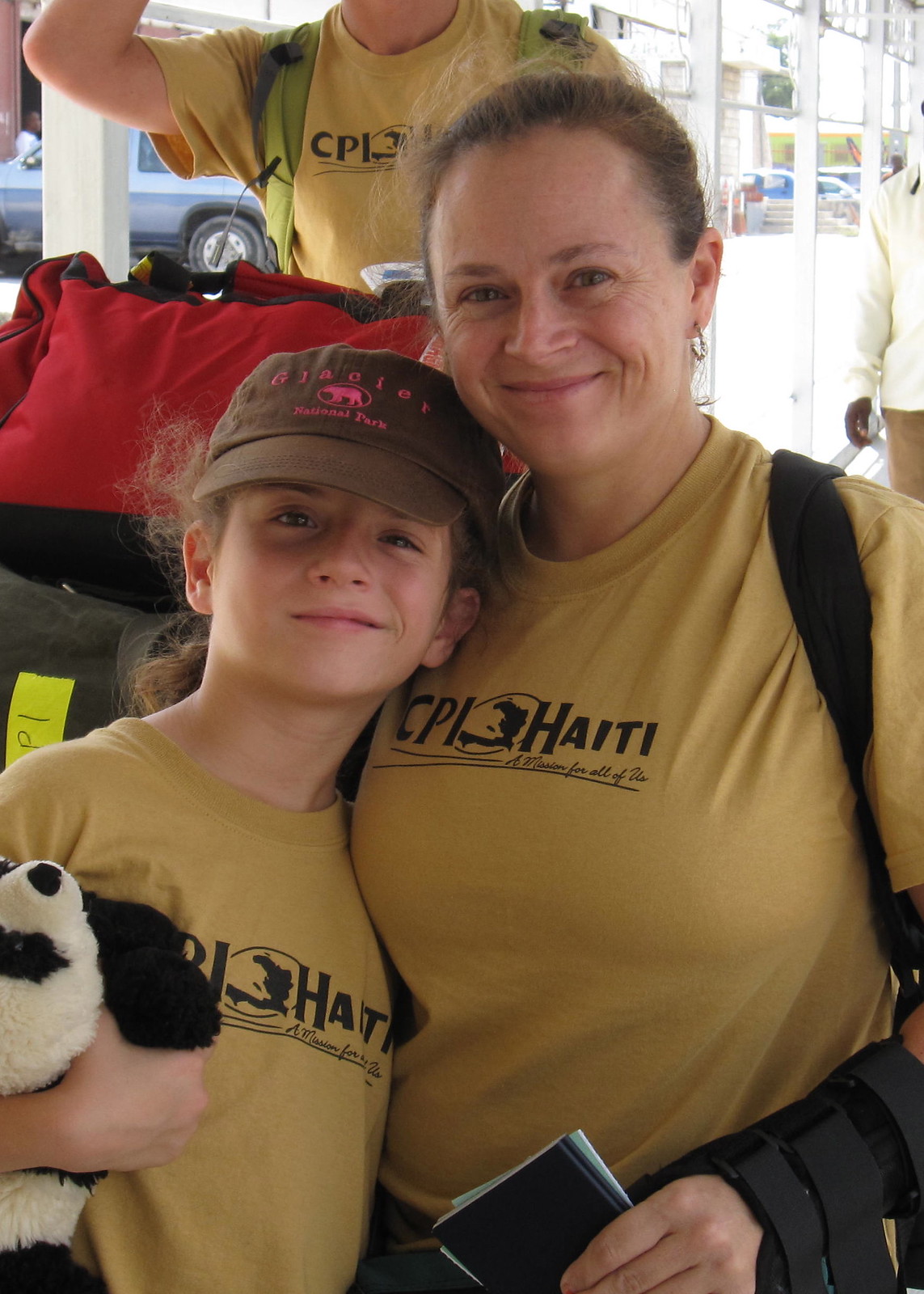A mother and daughter, likely on a mission trip, stand together in what appears to be a parking lot or breezeway. Both are dressed in brown T-shirts emblazoned with "CPI Haiti." The daughter, who is wearing a matching brown hat and holding a panda, stands close to her mother. The mother, with a wrist brace on her right arm, clutches some documents and has a bag slung over her shoulder. Behind them, another individual in a similar "CPI Haiti" T-shirt manages several pieces of luggage on a cart. Further in the background, another person, possibly African-American based on their hands, is seen walking. Multiple cars can be observed behind the group, suggesting they are preparing to depart or have just arrived. This evocative scene captures the camaraderie and anticipation typical of a group ready to embark on a communal journey or humanitarian effort.